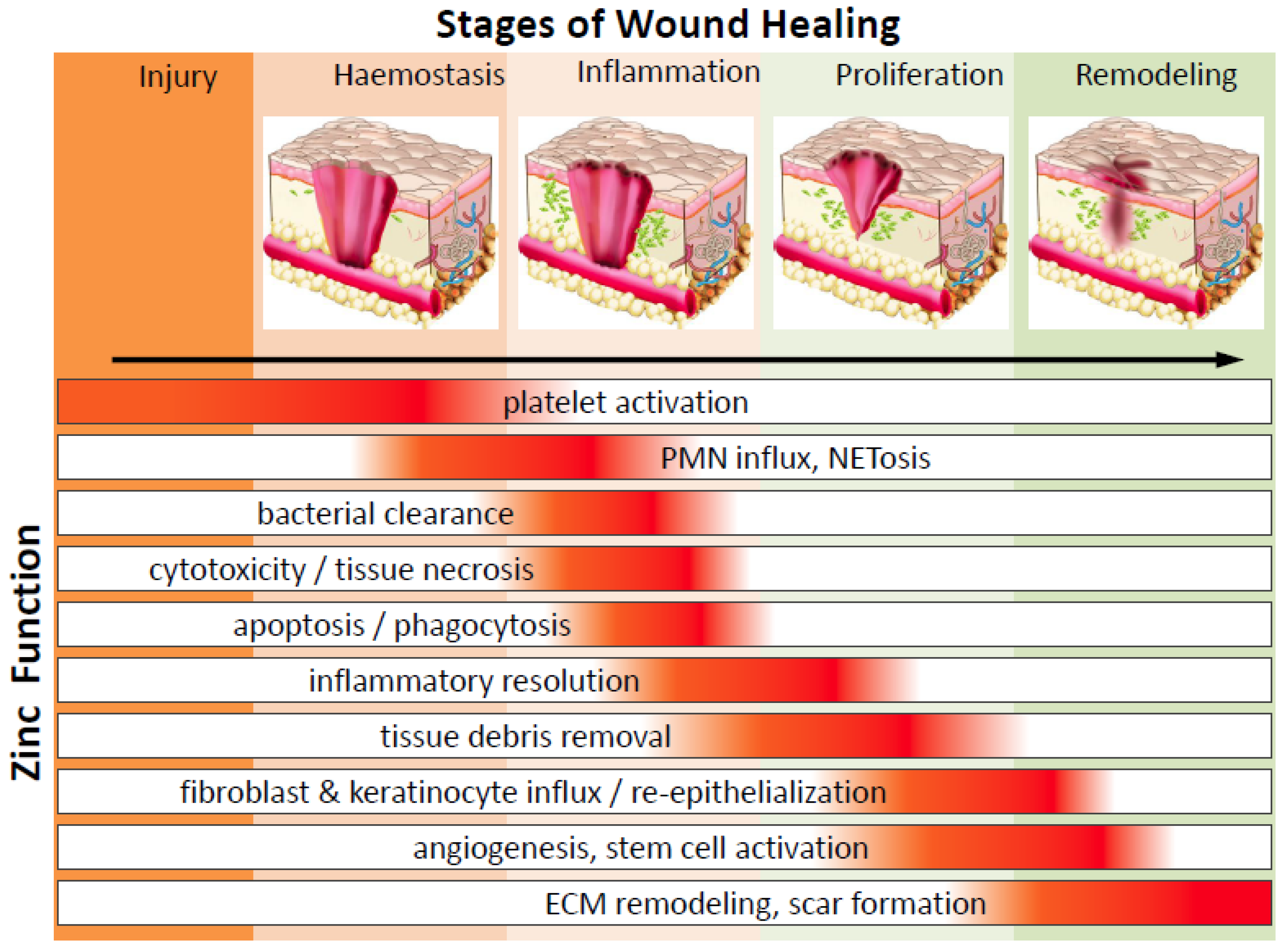The illustration, titled "Stages of Wound Healing," appears to be from a scientific textbook. At the top of the image is a sequence of cutaway diagrams illustrating the stages of wound healing, depicted in cross-sections of skin. The sequence begins with "Injury," represented by a plain orange block. This is followed by "Hemostasis" (British spelling: haemostasis), showing a side view of damaged tissue with a central wound depicted as a pink seashell shape, with red capillaries visible.

Next is the "Inflammation" stage, where the wound appears darker red and is covered by a browning, oozing substance, symbolizing the inflammatory response. Small green shapes near the wound indicate immune cells or other elements involved in the inflammatory process.

The "Proliferation" stage shows the wound beginning to close up, with the bottom healing and fewer green immune cells. Finally, in the "Remodeling" stage, the wound is almost entirely healed, leaving behind a minimal scar.

Beneath these images is a continuous black arrow running from left to right, labeled "Platelet Activation," which marks the progression of the healing process.

Below this arrow is a detailed chart titled "Zinc Function," resembling a bar graph. This chart lists various processes involved in wound healing: PMN influx and netosis, bacterial clearance, cytotoxicity/tissue necrosis, apoptosis/phagocytosis, inflammatory resolution, tissue debris removal, fibroblasts and keratinocyte influx, re-epithelialization, angiogenesis, stem cell activation, ECM remodeling, and scar formation. This chart visually complements the stages depicted above, providing a comprehensive overview of the cellular and molecular activities during wound healing.